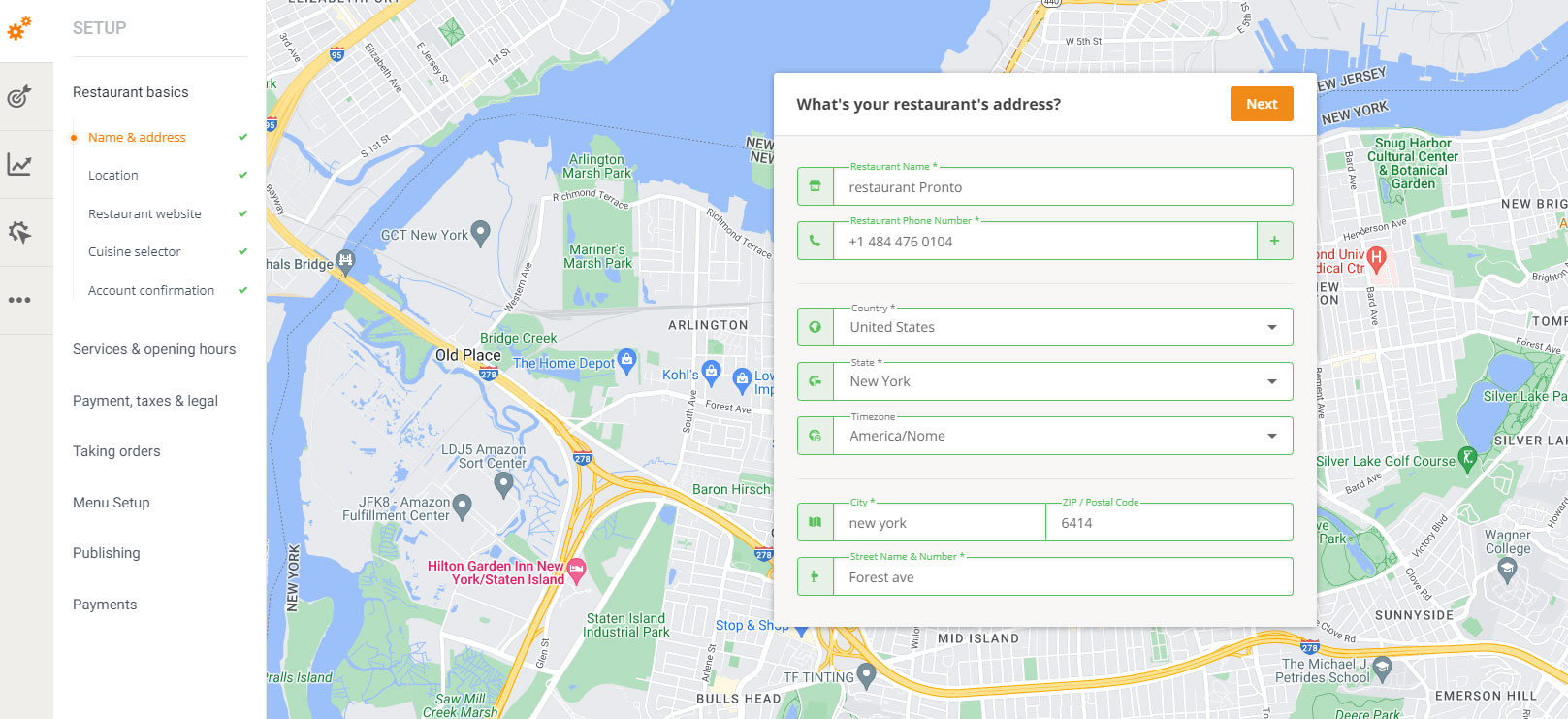This is a screenshot from a Maps application, showcasing a detailed setup interface. At the top left corner, a white header spans the width of the screen, featuring two orange cog icons on the left side. The smaller cog is positioned slightly to the right of the larger one. Next to these icons, in all caps light grey text, the word "SETUP" is displayed, underlined by a thin light grey line.

Beneath this header, there are two vertical sidebars. The leftmost sidebar is pale beige and contains four buttons at the top, each represented by a distinct dark grey icon, separated by thin horizontal grey lines. The top icon is a target with an arrow piercing through it, followed by a graph showing an upward trending arrow. The third icon looks like a sun with a cursor arrow on top of it, and the last one consists of three horizontally aligned dark grey dots.

The second sidebar, located to the right of the first, has a white background. At the top left corner, bold black text reads "RESTAURANT BASICS." A vertical thin light grey line runs underneath this text. Adjacent to this line, an orange circle holds the orange text, "NAME AND ADDRESS," which is accompanied by a green checkmark to its right. Continuing down the sidebar, similarly formatted entries appear with green checkmarks next to them, labeling "LOCATION," "RESTAURANT WEBSITE," "CUISINE SELECTOR," and "ACCOUNT CONFIRMATION." Below these labels, in larger dark grey text separated by ample white space, are additional categories: "SERVICES AND OPENING HOURS," "PAYMENT," "TAXES AND LEGAL," "TAKING ORDERS," "MENU SETUP," "PUBLISHING," and "PAYMENTS."

To the right of these sidebars, occupying the majority of the screen, is a large map image, showcasing the primary content area of the application.